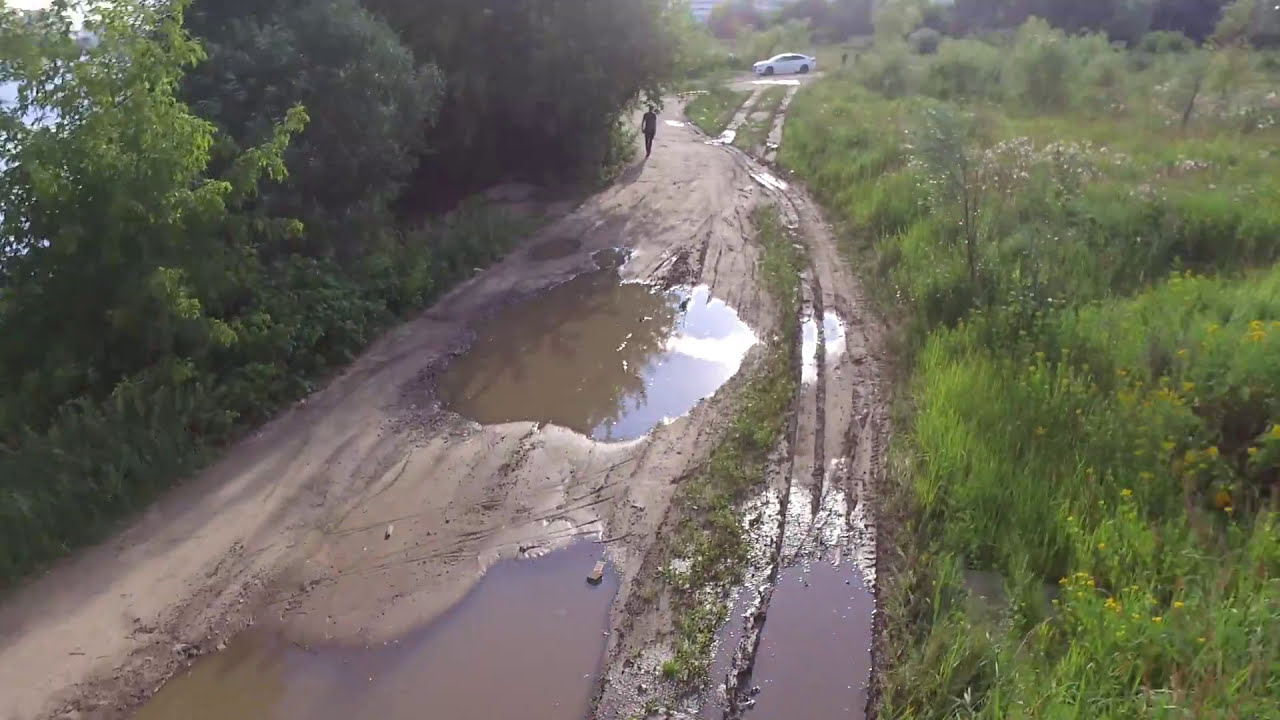The photograph captures a muddy dirt road, likely taken shortly after rain, with sizable brown puddles dotting its surface. On the right side of the road, there’s an assortment of slightly overgrown weeds, wildflowers, and small bushes, with some taller trees visible towards the top of the image, albeit blurred. On the left, dense bushes and taller trees obscure a body of water, hinting at a lake or similar landscape feature, barely visible through the foliage. The sky appears overcast, amplifying the wet and possibly tropical setting. A single silhouette of a person walks towards the camera, approximately a hundred feet away. Further down the road, a white four-door sedan is parked facing the water, with two individuals standing near its back. Tire marks weave around the puddles, indicating attempts to navigate the muddy terrain.